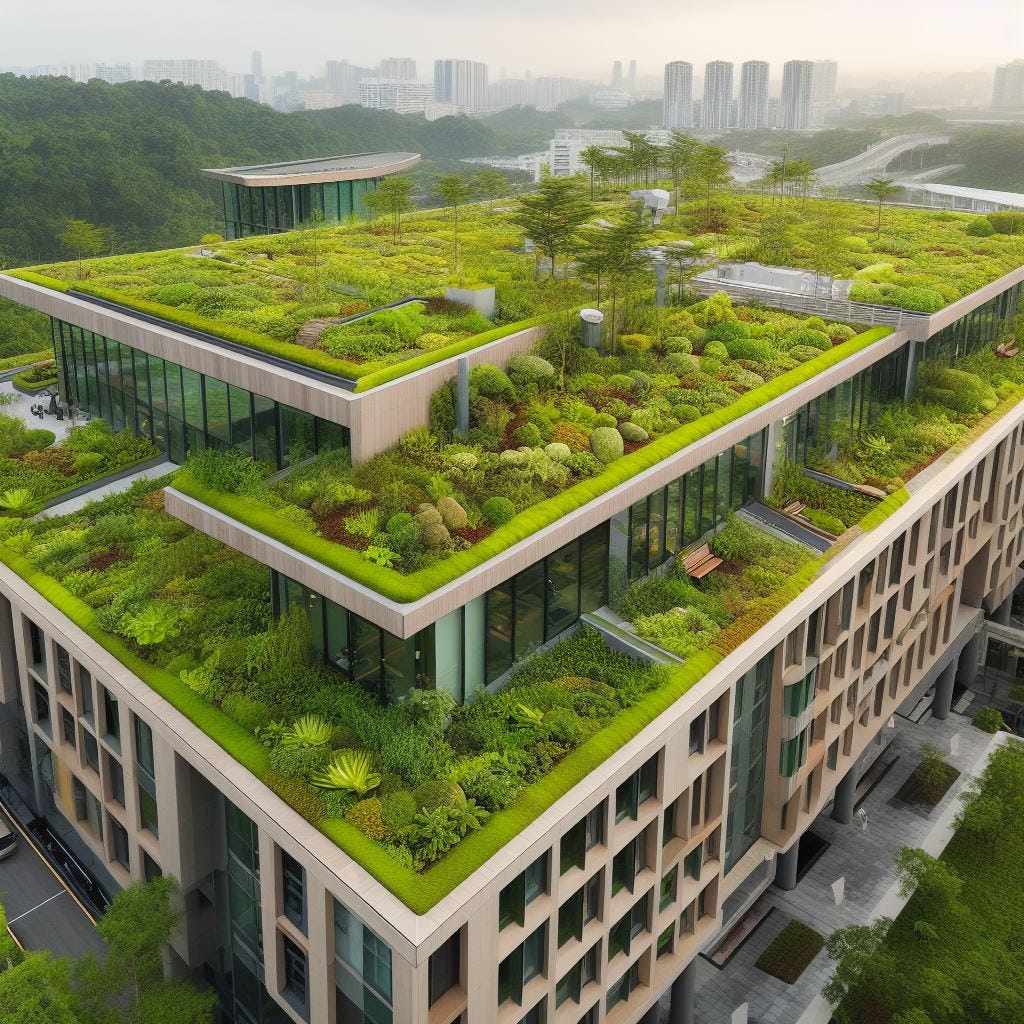This is an aerial, color photo of a modern, concrete building complex that appears to be around five stories high, slightly taller than it is wide, resembling a square in shape. The building has several distinctive layers: the first three floors feature numerous windows framed in concrete, reminiscent of an office space or possibly a large apartment complex. The building’s facade is predominantly beige-gray with green shutters around the windows. 

Atop the third floor, the building transforms into a verdant oasis. The fourth floor features an expansive garden with green plants, succulents, various shrubs, and an outside bench facing outward, creating a green eco-friendly space. This continues up to the fifth floor and final rooftop, which is layered and filled with more greenery, including small palm-like trees and various other vibrant plants, creating a lush, multi-level garden. 

The photo further captures a gray concrete sidewalk with visible columns supporting the building. The surrounding background shows a hazy city skyline with tall skyscrapers under a cloudy, light-gray sky, adding an urban context to the scene.